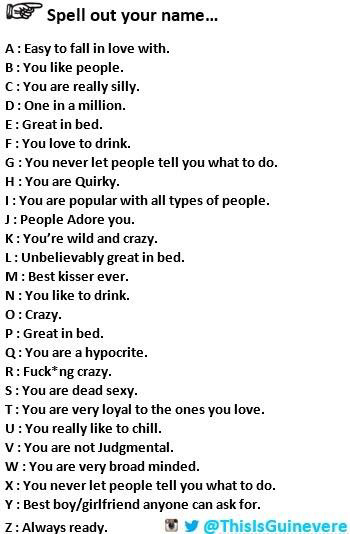This is an online image featuring a list titled "Spell Out Your Name," accompanied by a pencil drawing of a hand with a finger pointing to the left. The list runs vertically from A to Z, with each letter corresponding to specific personality traits. The descriptions are as follows: A - easy to fall in love with, B - you like people, C - you're really silly, D - one in a million, E - great in bed, F - you love to drink, G - you never let people tell you what to do, H - you are quirky, I - you are popular with all types of people, J - people adore you, K - you're wild and crazy, L - unbelievably great in bed, M - best kisser ever, N - you like to drink, O - crazy, P - great in bed, Q - you are a hypocrite, R - effing crazy, S - you're dead sexy, T - you're very loyal to the ones you love, U - you really like to chill, V - not included, W - you're very broad-minded and never let people tell you what to do, X - not included, Y - not included, Z - always ready. The bottom right corner features social media handles @thisisguinevere in blue, alongside Instagram and Twitter logos. The image serves as a playful online game where individuals spell out their names to match the corresponding traits, often used for light-hearted entertainment.